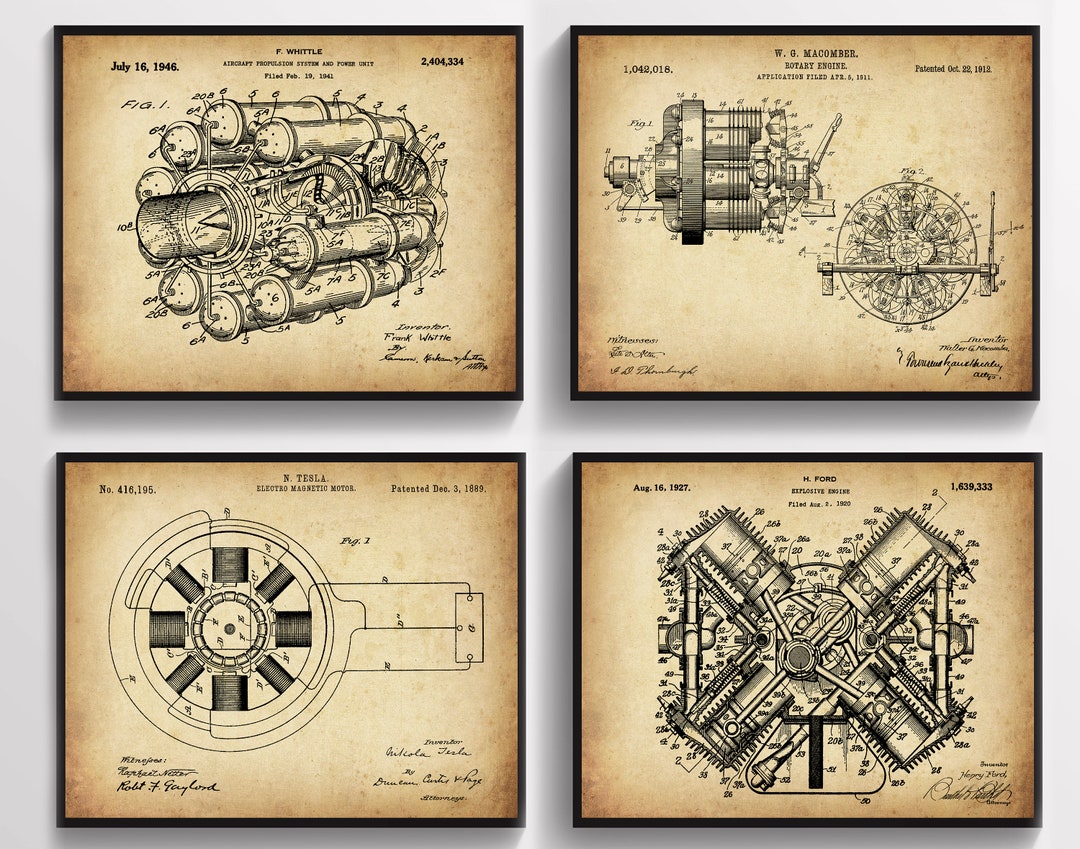This image features four framed, antique-style diagrams set against a wall in a uniform display, each encased in a thin black frame. The paper within each frame has a brownish-white, aged appearance, reminiscent of historical documents like the Constitution. Each diagram includes text and various technical illustrations, though some of the text is difficult to decipher. The diagrams are arranged in a grid with two on top and two on the bottom.

Starting from the top left, the first diagram is dated July 16, 1946, titled "Aircraft Propulsion System and Power Unit" by inventor Frank Whittle, identified by patent number 2,404-334. The illustration details what appears to be a complex system of interconnected tubes and mechanisms, labeled and annotated with small text.

The top right diagram, attributed to W. G. Macomber, is labeled "Rotary Engine." It includes multiple views of the engine, both in profile and head-on, showcasing various tubes and mechanical parts.

In the bottom left is a diagram titled "Electric Magnetic Motor" by N. Tesla. This schematic outlines the internal components of a motor, marked with various numbers and letters.

The final diagram, in the bottom right, is labeled "Explosive Engine" by H. Ford. It provides an intricate view of an early engine design, possibly intended for one of Ford’s early automobiles, with detailed components and annotations.

Together, these illustrations present a fascinating glimpse into the technical innovations of notable inventors from the past, with each diagram offering a detailed, though partly obscured, view of groundbreaking mechanical designs.